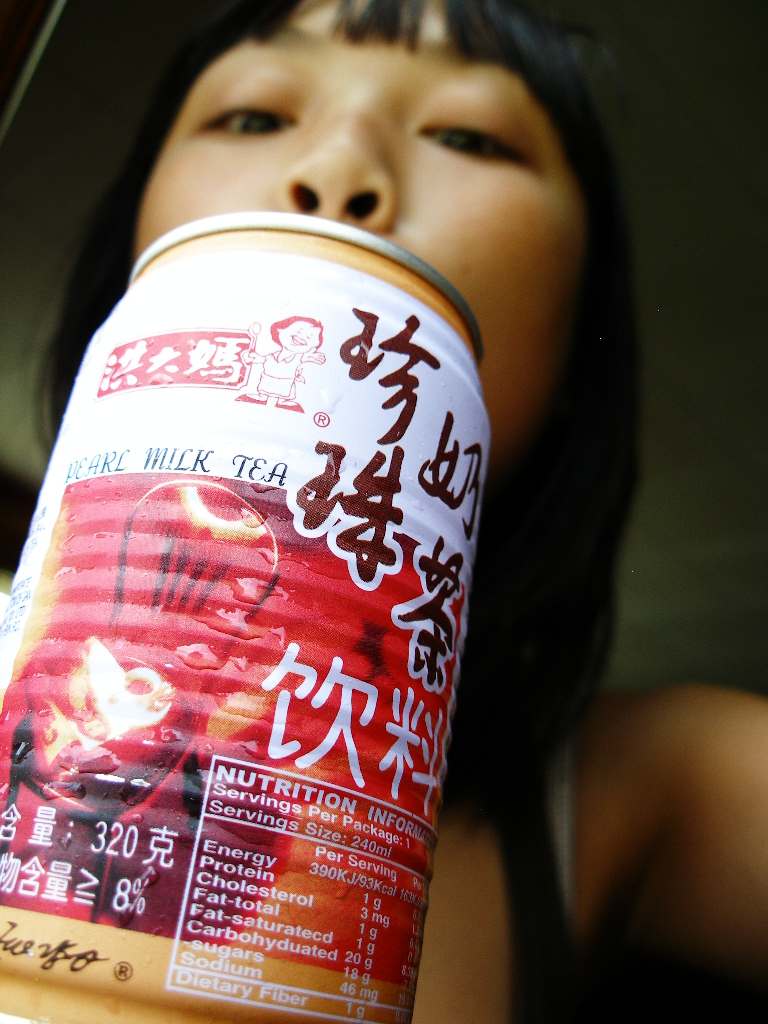In this captivating photo, an Asian woman with black, shoulder-length hair and blunt bangs is holding a can of pearl milk tea. The viewer's perspective is from below, looking up at her as she gazes downward, her face partly visible above and behind the can. The woman has brownish-yellow skin and her expression is focused on the camera lens.

The can itself prominently features a vibrant red background towards the bottom, with the text "pearl milk tea" clearly displayed. The upper left corner of the can boasts an illustration of a woman in an apron holding a spoon, with adjacent Asian characters adding to its authentic appeal. The illustration of the woman, who appears to be an endearing 'Asian mom' figure, is enclosed in a red box on the can, which also includes the nutrition facts in a white section. The overall design merges traditional Asian elements with a modern beverage, making the can both visually and culturally striking.